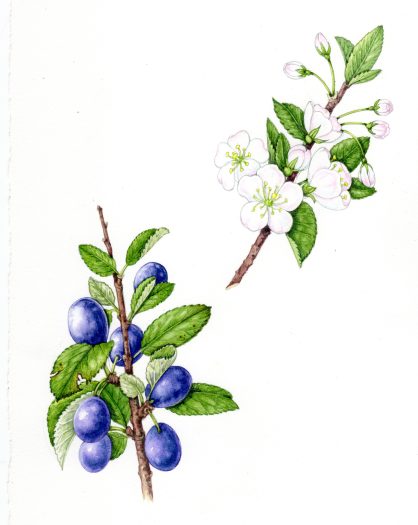This image is a detailed drawing on a white background, accentuating the colors of the depicted plants. There are two main branches in the composition. The branch in the lower left corner features a thin, brown stem with green leaves and seven round, dark blue fruits resembling blueberries. The branch on the top right displays delicate white flowers with five petals each, surrounding a green center adorned with fine yellow stamens. Alongside the blooms are five additional buds yet to open. Both branches share similar stems and leaves, suggesting they may belong to the same plant species, showcased against a pristine white backdrop to emphasize their vibrant colors and intricate details.